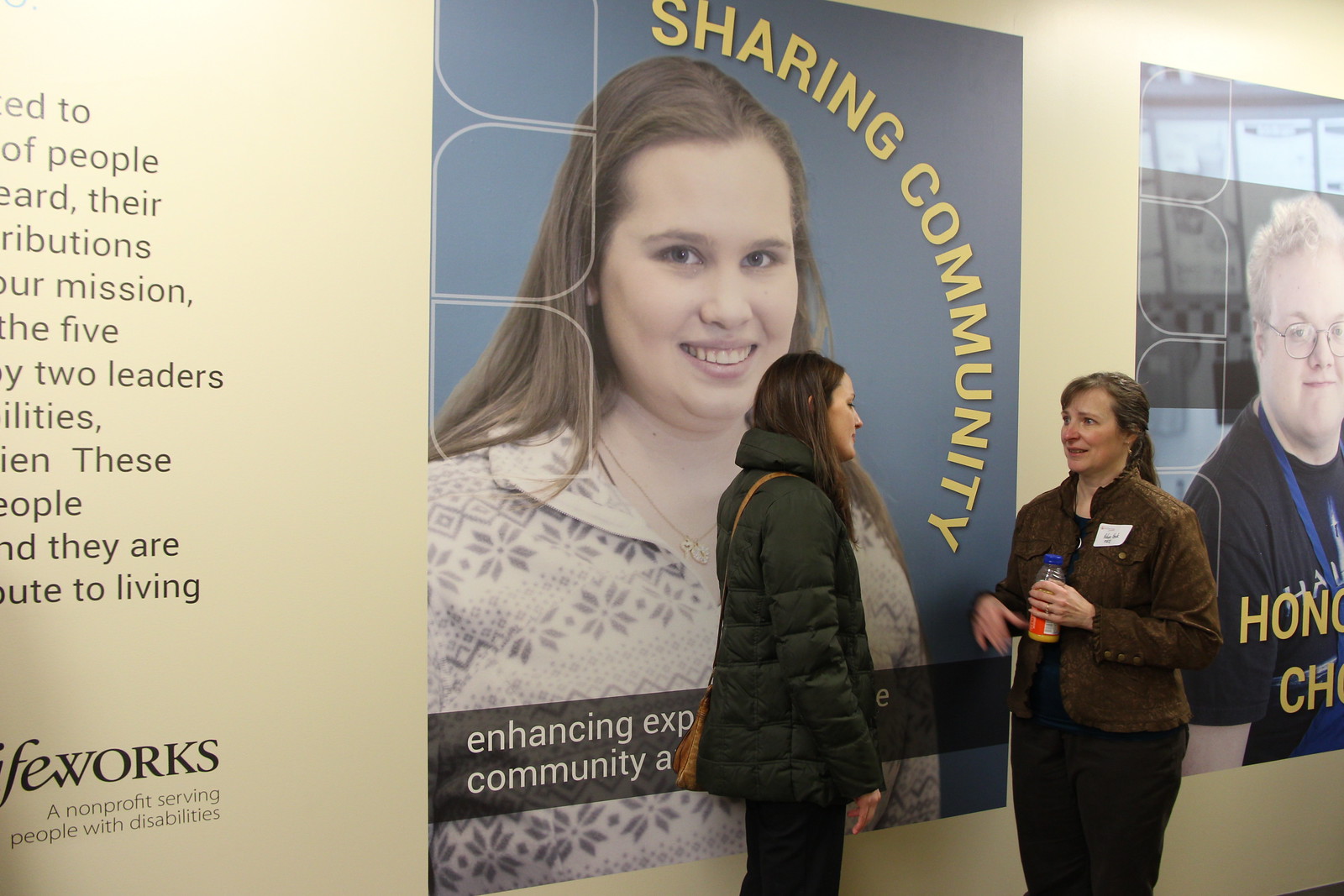The photograph shows two women engaged in conversation, standing sideways to the camera. The woman on the left is donning a black puffer jacket, dark hair, and a brown crossbody purse, facing the right. The woman on the right is captured mid-motion, holding a bottle of orange juice with a blue cap. She has dark hair styled in low ponytails, a flush Caucasian face with red cheeks and nose, and is wearing a brown jacket over a dark blue t-shirt with dark brown pants. They stand before a beige background adorned with two large posters. The left poster, against a blue background, features a smiling woman in a white fleece jacket with a gray snowflake print, accompanied by yellow text that reads "sharing community." Adjacent to it, partially visible, is another poster depicting a man with blonde hair, wearing glasses and a black t-shirt with a blue lanyard. This poster includes cropped yellow text starting with "H-O-N-O" and another fragment beginning with "C-H." The scene suggests a professional or community event, potentially an expo, with the woman holding the juice bottle also wearing a name tag, implying a semblance of formal interaction or introduction.